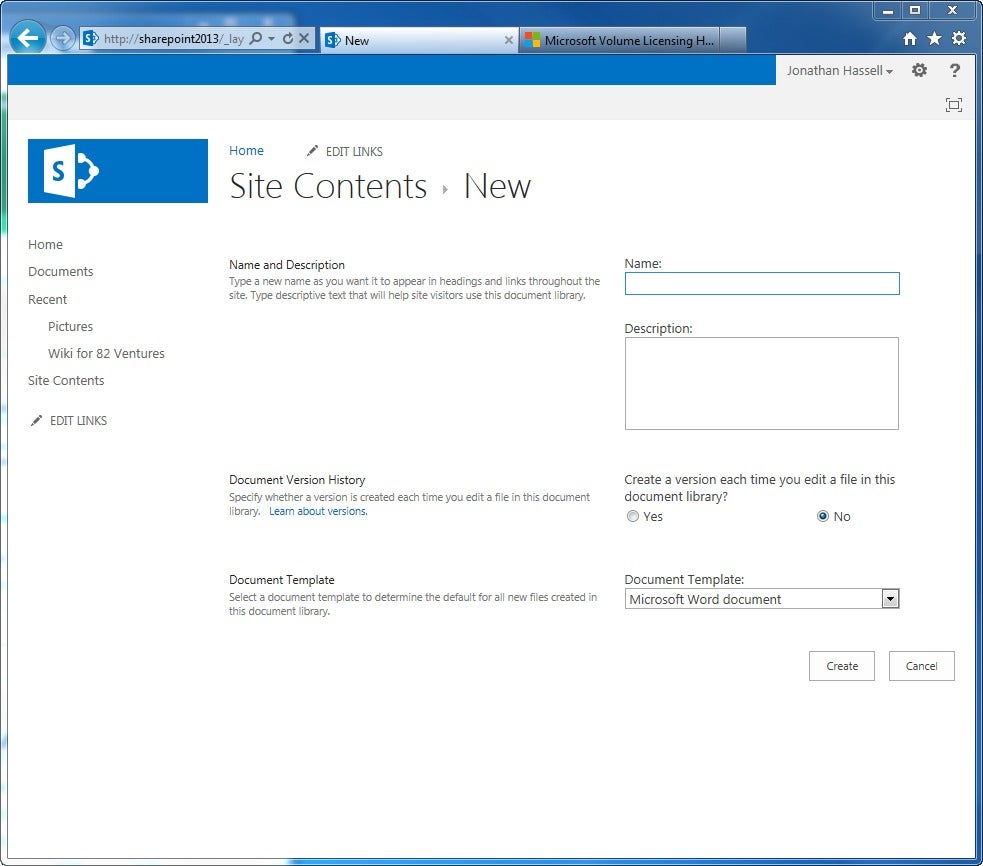Screenshot of a web page displaying various browser and website elements. The browser interface includes a back arrow, URL bar, new tab button, and tabs for Microsoft and other sites. Browser window controls such as minimize, maximize, and exit are visible at the top right corner. Within the webpage, there are icons and buttons for home, favorites (star icon), settings, and help (question mark). There are sections labeled "Home," "Document," "Reward," and "Pictures."

Additionally, the site appears to be related to a wiki for "82 Ventures," featuring options for site context, edit functions, and navigation tabs such as "UNS" and "UMS." The editing interface includes fields for "Name" and "Description," alongside options to create or cancel. A blue border highlights interactive elements on the screen. Circles labeled "No" and "Yes" likely represent selection buttons for user choices.